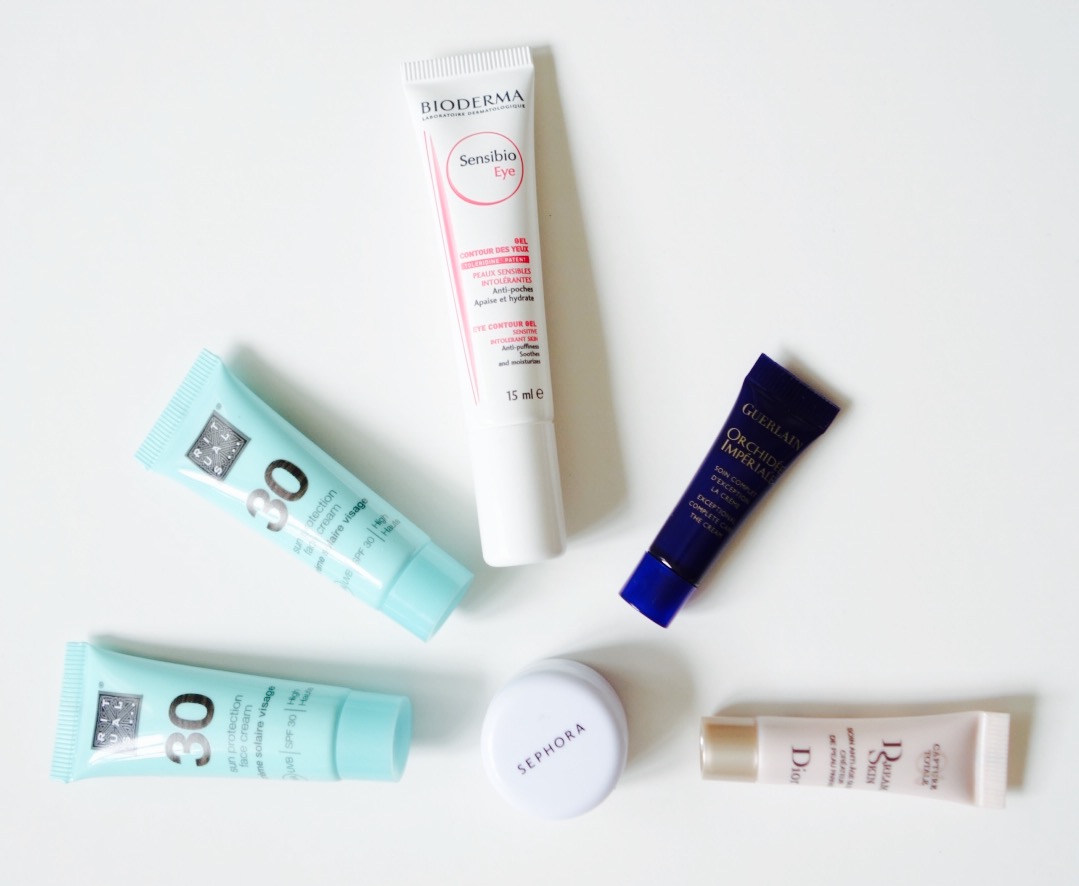The image showcases an assortment of cosmetic products meticulously arranged on a white background. Central to the composition is a small, round, white container labeled "Sephora" in elegant black lettering. This container, likely made of either porcelain or plastic and featuring a screw-top lid, is positioned at the center bottom of the arrangement. 

To the container's right, at approximately the three o'clock position, sits a light cream-colored tube with a gold cap, oriented such that the cap faces the Sephora container. This tube, a product by Dior, is labeled "Radiant Skin" with writing in a delicate burgundy or brown hue.

Moving clockwise to the 1:30 position, there is a dark blue tube topped with a royal blue cap, also positioned cap-down towards the Sephora container. This tube features gold lettering that reads "Crypsis Imperial."

Near the 12 o'clock position, slightly left of center, is a white tube with a white cap. The capped end of this tube is ridged, and it bears the brand name "Bioderma," along with the product name "Sensibio Eye." The tube is accented with a red stripe on the left side and a red circle containing the product name. It is described to have 15 milliliters of product, with additional red and black text.

At approximately the 10 o'clock position is an aqua blue tube with a matching cap. This item, from the brand Rituals, is identified by the label "RITUALS..." rendered in black text. The product appears to be a sun protection skin cream, with "30" possibly indicating the SPF value.

Finally, positioned at the nine o'clock mark is another aqua blue tube, identical to the one found at the 10 o'clock position, completing the circle of products.